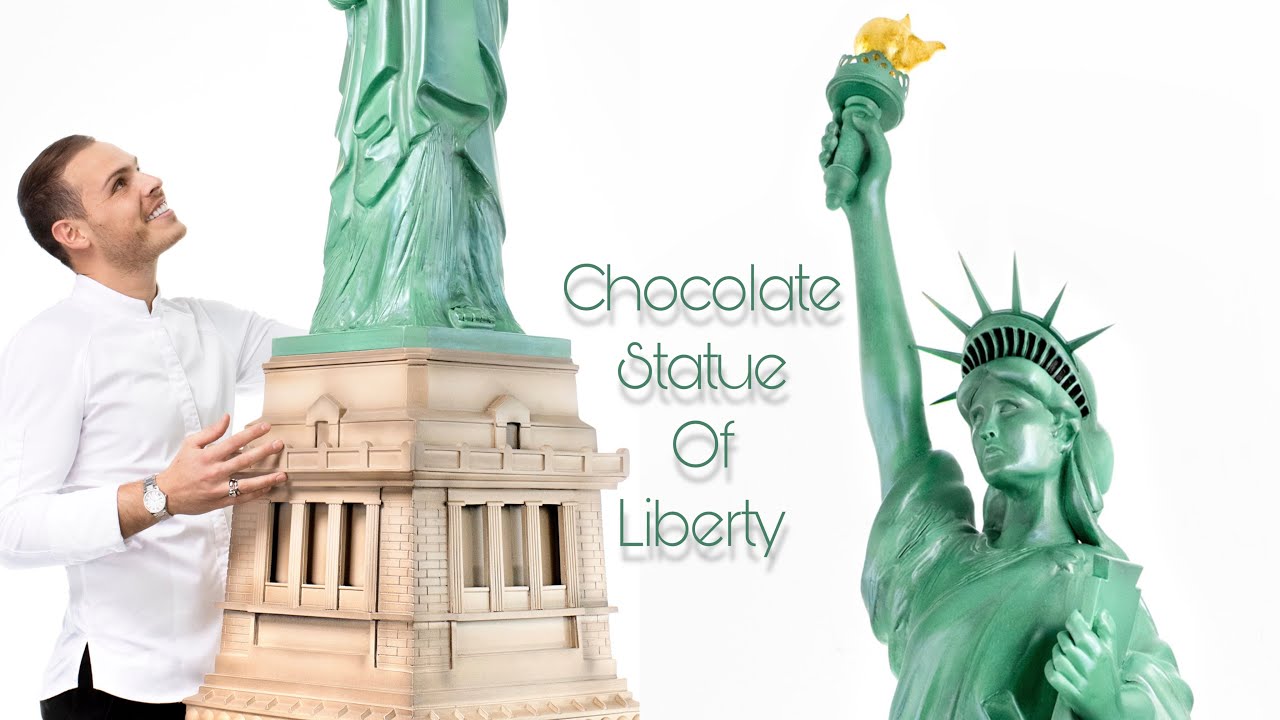This image showcases a striking and imaginative display titled "Chocolate Statue of Liberty," indicated by green, shadowed text at the center against a white background. It features the Statue of Liberty seemingly cut into two parts: the left side shows a man in white chef attire, black trousers, a silver watch, and a ring, grinning as he looks up at the statue's skirt while holding its tan stone-like base. On the right, the upper portion of the green-hued Statue of Liberty holds up the book and torch, with intricate detailing, including the torch’s yellow flame, suggesting a life-size rendition. Despite its green appearance reminiscent of the original statue, the claim is that it’s crafted entirely from chocolate, adding to the extraordinary nature of the artwork.